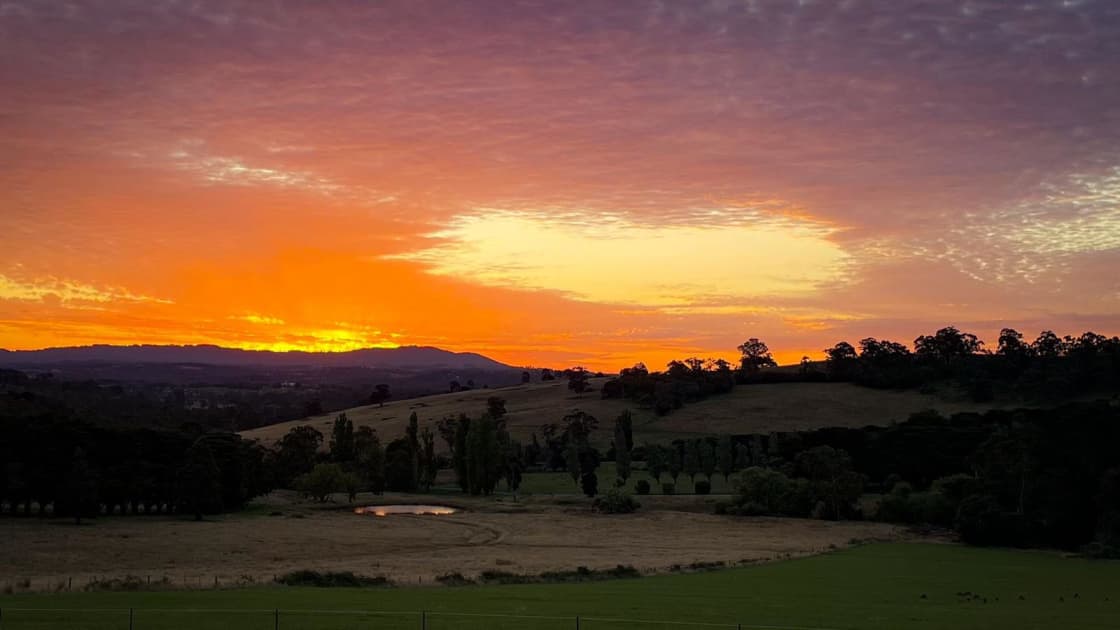An enchanting landscape scene depicted in either a photograph or a highly realistic painting, showcasing the beauty of dusk, or possibly dawn, over a serene valley. The sky is a vibrant tapestry, transitioning seamlessly from deep orange near the horizon to soft pink, lavender, and dusky bluish-purple tones higher up, reminiscent of a rainbow. Majestic, gently sloping hills and mountains bathed in rich, cool green and purple hues form the horizon. The foreground features a lush patch of bright green grass, almost glowing in the fading light. Scattered trees and shrubbery populate the landscape, with denser clusters on the left and right. A tranquil pond, reflecting the brilliant oranges of the sky, sits in the valley surrounded by patches of darker grass. Wisps of lavender and purple clouds hang in the sky, adding to its ethereal beauty. There are distant houses, suggesting a sparsely populated, idyllic farming community. The entire scene exudes a surreal, almost otherworldly charm, heightened by the warm light of the setting (or rising) sun.